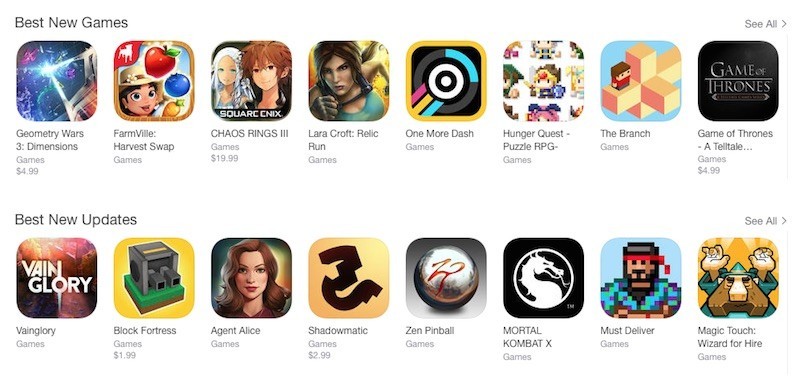In this image, we see a section from a website or mobile application showcasing the latest game offerings. The background is white, providing a clean and minimalistic look. In the top-left corner, there is a header titled "Best New Games." On the top-right corner, a "See All" tab is available for users wishing to view the entire list of new games.

Below the header, several game suggestions are neatly arranged in tiles, each displaying the game's name. The featured games include "Geometry Wars 3," "Farmville: Harvest Swap," "Chaos Rings 3," "Lara Croft: Relic Run," "One More Dash," "A Hungry Quest: Puzzle RPG," "The Branch," and "Game of Thrones."

Continuing downward, there is another section titled "Best New Updates." This section showcases games that have recently received significant updates. The listed games are "Vainglory," "Black Fortress," "Agent Alice," "Shadowmatic," "Zen Pinball," "Mortal Kombat X," "Must Deliver," and "Magic Touch: Wizard for Hire." There is also a "See All" button above the last application in this section, allowing users to explore more updated games.